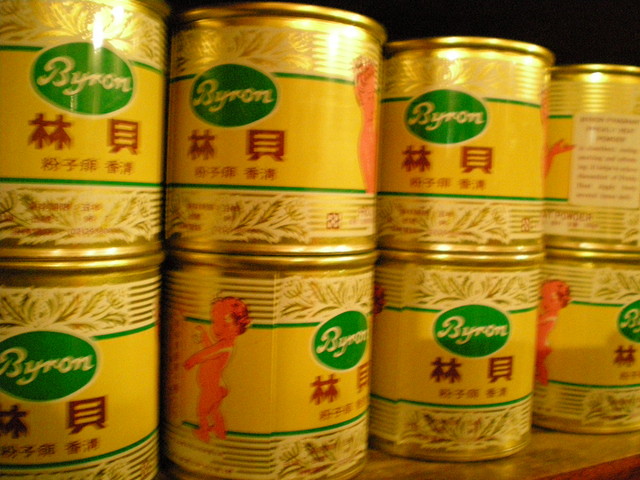The image displays eight cans, each adorned with distinctive Asian-themed labels. Central to the label's design is an oblong, rounded tag bearing the name "Byron" in prominent white lettering. Below "Byron," there are two larger Asian symbols followed by a row of approximately five smaller Asian characters. Beneath these characters, a decorative floral pattern enhances the aesthetic appeal.

Notably, a few cans are positioned to reveal an illustration of a nude infant or child holding a white flower, which suggests the possibility that these are containers of jasmine tea, known for its floral notes. However, it is not entirely clear if they contain tea or another type of product. The intricate and culturally rich design hints at the product's Asian origin, adding an element of authenticity and allure to its presentation.